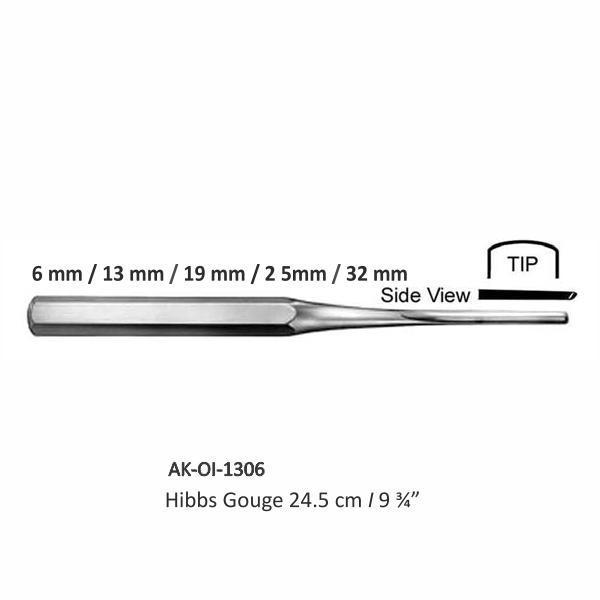The image, set against a white background, displays a diagram of a small tool resembling a gouge or a modified screwdriver. The tool is silver in color, horizontally aligned with the tip facing right. It features a hexagonal base that tapers to a fine, rounded tip. Above the tool, in black text, are the measurements: "6mm / 13mm / 19mm / 25mm / 32mm." Next to these measurements, on the right, is the word "side view" followed by a detailed illustration of the tool's tip, labeled "TIP" in all caps. Below the main image, in bold black letters, are the inscriptions: "AK-01-1306" followed by "Hibbs gouge 24.5cm / 9.75 inches."